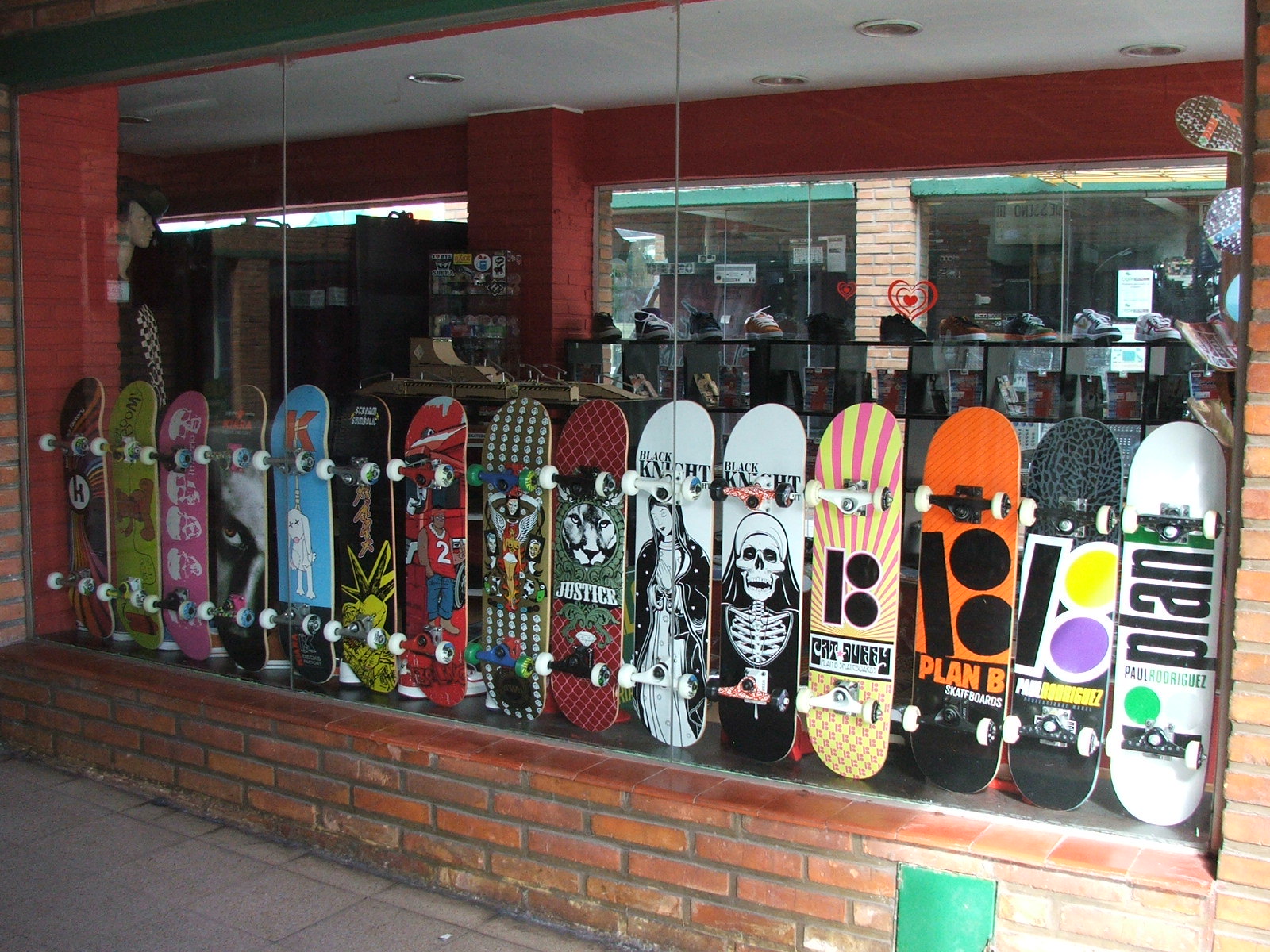In this photograph of a storefront, the camera captures the exterior of a red brick building with a large, three-pane glass window prominently displaying an array of colorful skateboards. Propped vertically with their white wheels pressed against the glass, the skateboards immediately draw attention to the varied and vibrant designs. Adorning the boards are graphics such as white skulls on a pink deck, a nun with a skeletal face, and depictions of the Virgin Mary and a lion. Specific boards feature text, including a white one that says 'Plan B', an orange and black one with the same label, and a textured gray skateboard that reads 'Paul Rodriguez'. The storefront's surroundings include a tiled cement sidewalk with clear lines and squares, and above the window is a green awning. Inside the store, visible through the window, there is a red-painted brick wall which enhances the vibrant atmosphere, contrasted by the white ceiling above. A heart sticker is discreetly placed on the glass, adding a personal touch to the scene.